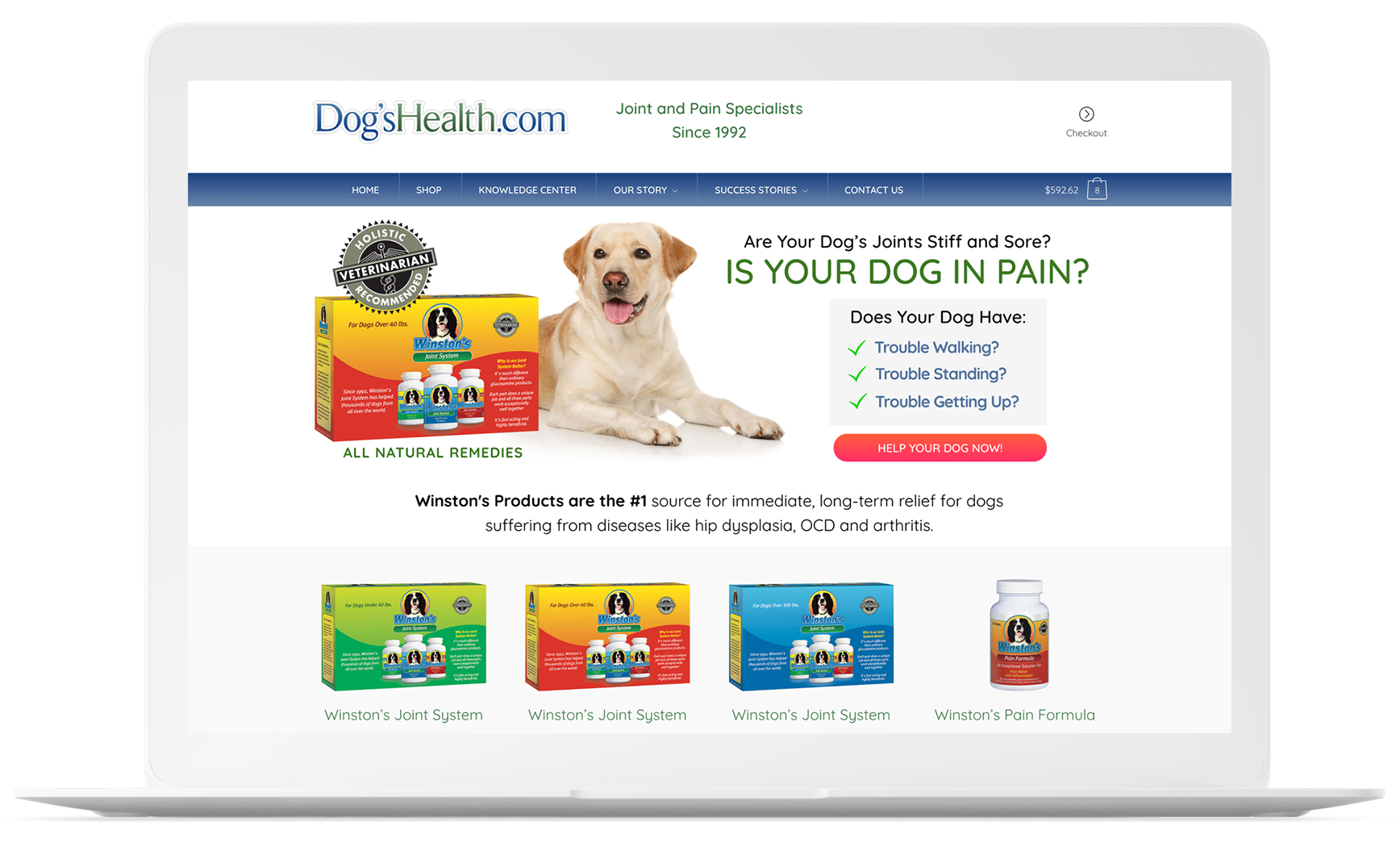The image depicts a laptop with a grey casing, screen open, displaying a website page with a white background. In the upper left-hand corner of the page, the URL "dogshelp.com" is prominently featured; "dogs" and ".com" are in blue, while "help" is in green. To the right, the site tagline "Joint and Pain Specialist Since 1992" is displayed in green text. On the far right, there is a circular icon with a right arrow and the word "Checkout."

Below this, a blue navigation banner includes links to "Home," "Shop," "Knowledge Center," "Our Story," "Success Stories," "Contact Us," and an unreadable dollar amount next to a shopping bag icon. 

Further down, a seal proclaiming "Holistic Veterinary Recommendation" overlaps a yellow and red box. This box features an image of a dog above three jars that also bear the same dog's image. Beside this box, a yellow Labrador Retriever is seated. 

Adjacent to the dog, black text asks, "Are your dog's joints stiff and sore?" followed by larger green text declaring, "Is your dog in pain?" Below this, a grey box lists symptoms with green checkmarks: "Trouble walking," "Trouble standing," and "Trouble getting up."